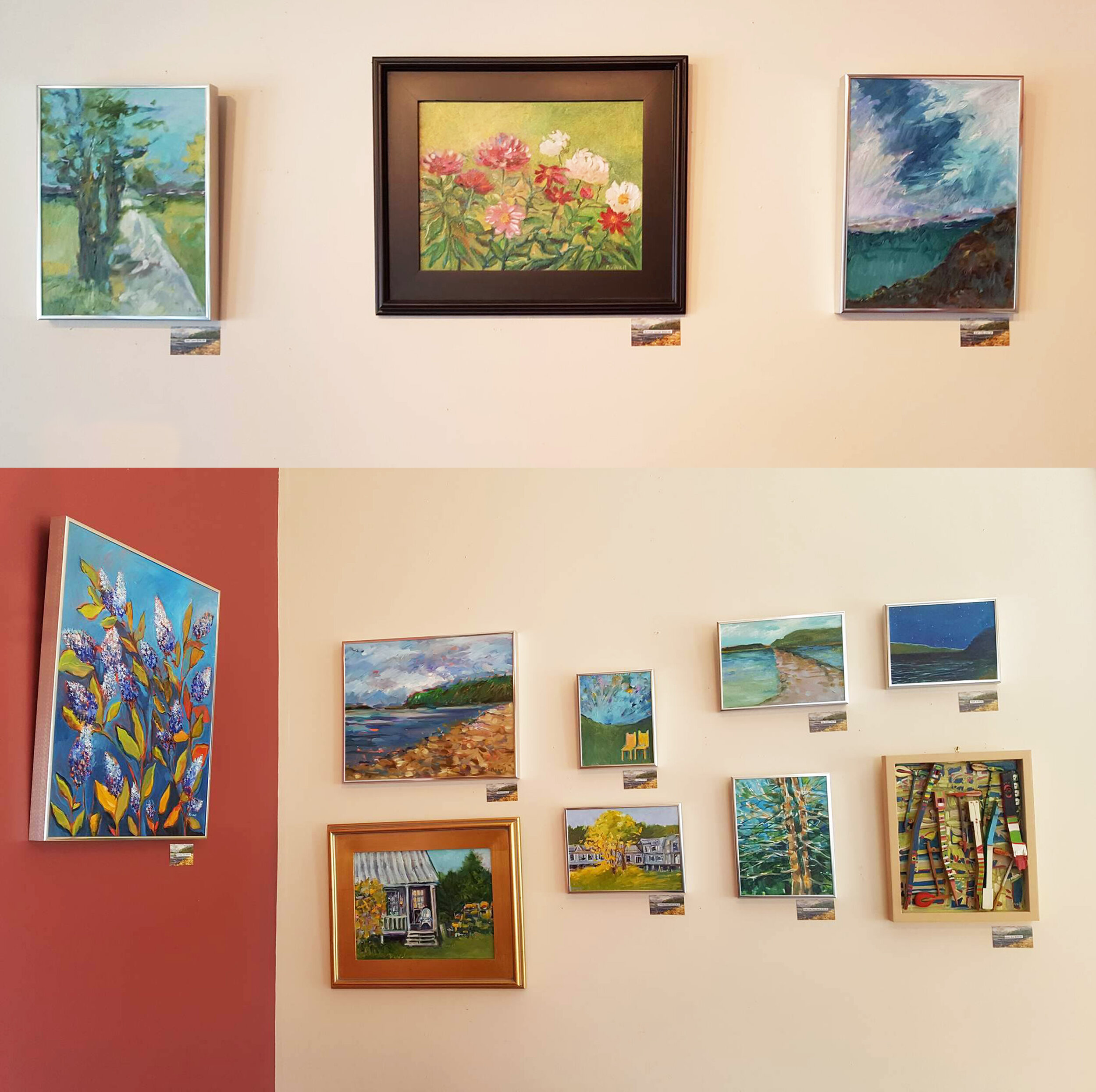The photograph features two sections of an art gallery wall, both dominated by light peach-colored tones, resembling the shade of Caucasian flesh. The upper section showcases three framed paintings, while the lower section displays eight. The artworks, which include scenes of nature such as flowers, trees, the ocean, a beach, a house, an outdoor pathway, a marsh, and leaves, exude a mix of amateur and elegant qualities. The left side of the lower image transitions from the peach hue to a dark red brick color, where a blue and green floral painting is positioned. The overall display suggests the paintings are for sale, adding a commercial dimension to the gallery setting.